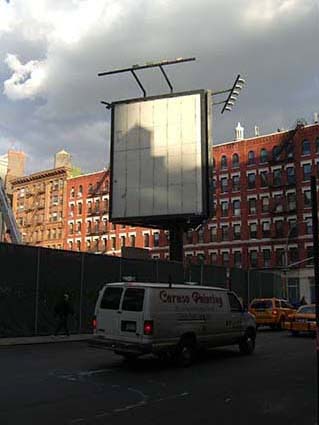This detailed urban photograph captures a bustling cityscape. In the foreground, a busy street is lined with vehicles; most notably, a white van with red writing on it, and two yellow taxis parked in front of it. The white van's brake lights are on, indicating it may be preparing to move. To the left of the street, a gray sidewalk hosts a gentleman walking, and another individual is visible near the taxis. Adjacent to the sidewalk, a towering ten-foot-tall fence draped with green mesh divides the sidewalk from a significant structure in the background.

Dominating the left and central portions of the image, this fence separates the hustle and bustle of the street from the substantial and somewhat mysterious structure behind it, resembling a hybrid between a solar panel array and a lighting installation. Farther behind this, a large red-brick building with white trim extends across almost the entire background, indicative of either offices or apartments, mirroring the architectural style typical in Manhattan, New York City. Some sections of the building display light tan-brown bricks.

Overhead, the sky is partially filled with bright, white clouds, with a hint of grayish-blue peeking through at the top left corner, portending an incoming storm. A prominent white tower rises in the background, adding vertical interest to the scene. Additionally, a vertical, rectangular sign with a black frame and white face stands out among the urban elements, further emphasizing the city's dynamic environment.